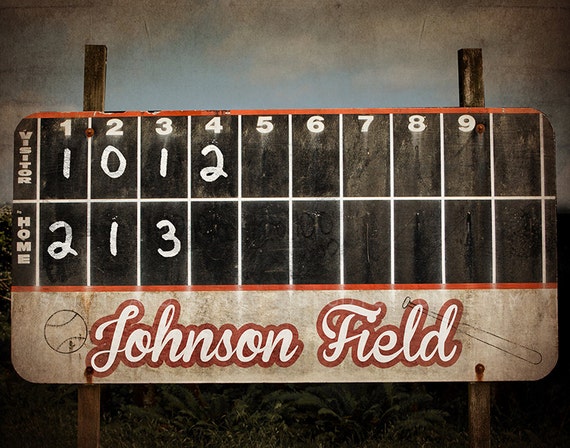The square, full-color photograph depicts a vintage baseball scoreboard set outdoors under natural light. The scoreboard, rectangular in shape and supported by two posts, prominently displays the scores of a game currently in the bottom of the fourth inning. The visitors have accrued four points, with one in the first inning, zero in the second, one in the third, and two in the fourth. The home team leads with six points, having scored two in the first inning, one in the second, and three in the third. The backdrop of the scene is a partially overcast sky with patches of blue, and the base of the scoreboard is adorned with some ferns and foliage. Inscribed in cursive red lettering at the bottom of the scoreboard is "Johnson Field." A white border surrounds the scoreboard, which features a baseball motif and a bat graphic pointing downward to the right.